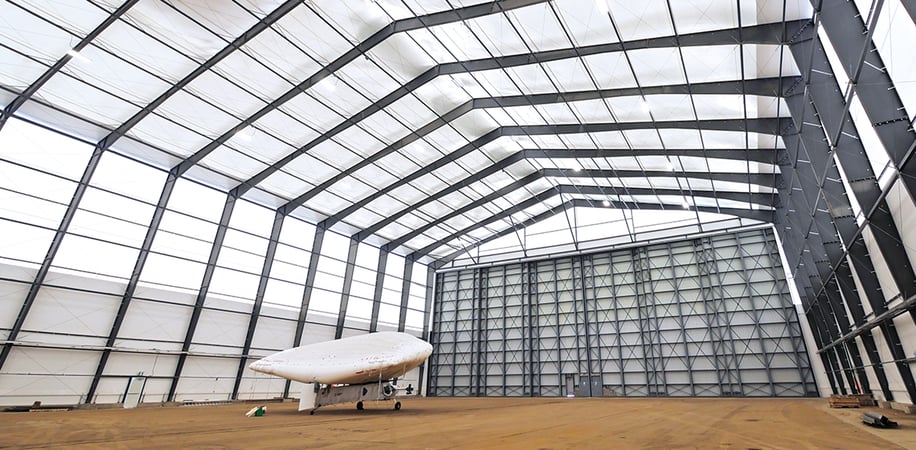The image depicts the interior of a large aircraft hangar constructed from light-permissive fiberglass panels supported by gray metal girders. The towering structure features a spacious, well-lit interior thanks to the translucent panels that allow ample natural light to permeate. The hangar's floor appears to be covered in dirt, contributing to its utilitarian appearance.

Centrally located within this expansive space is a single white object, likely an aircraft or drone with folding wings that align along the rear of its fuselage. This piece of machinery sits on wheels and may be jet-powered, although a propeller is not visible. Positioned towards the right side of the scene, the building's massive entryway is characterized by two large doors, appearing as a gateway for substantial aircraft. Overall, the hangar is predominantly empty, emphasizing its vast size and capacity for housing large vehicles or machinery.